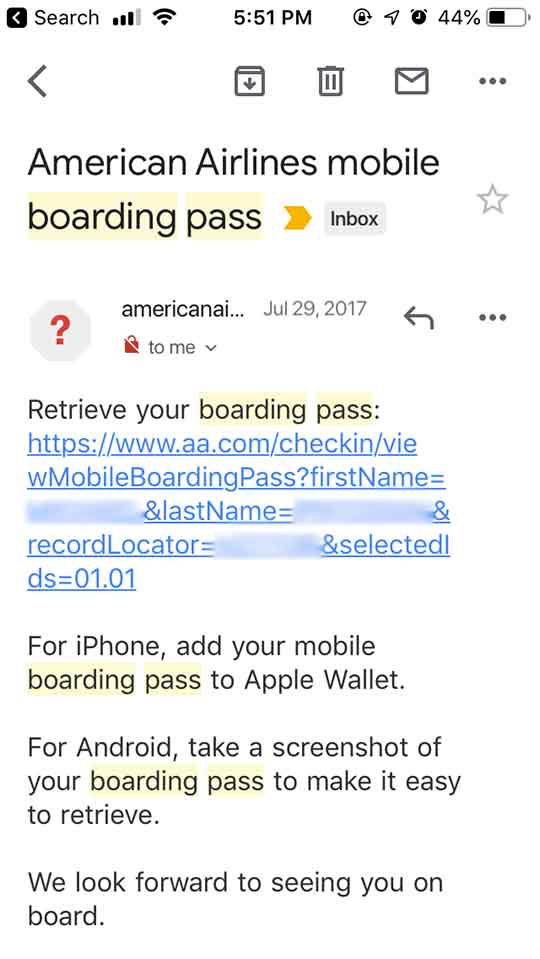The image is a detailed screenshot captured on a smartphone, showcasing an email interface against a white background. At the top left of the screenshot, black text reads "search" with a left-pointing arrow adjacent to it. Following this, there are icons indicating the cellular signal strength and Wi-Fi signal strength. Centrally located at the top, the current time is displayed as 5:51 p.m. To the far right, icons show the battery percentage and the screen lock status.

Directly beneath this top bar, another left-pointing arrow is visible on the left-hand side, accompanied by several icons including one for trashing the message and another for forwarding it. This further suggests that the screenshot is of an email interface. 

The email's tagline reads "American Airlines mobile boarding pass," indicating the sender is American Airlines and it is addressed to the recipient. The main subject of the email is "Retrieve your boarding pass," and it contains a link to access the boarding pass from American Airlines. Additional email content provides instructions for different phone users: "For iPhone, add your mobile boarding pass to Apple Wallet. For Android, take a screenshot of your boarding pass to make it easy to retrieve." The email concludes with, "We look forward to seeing you on board."